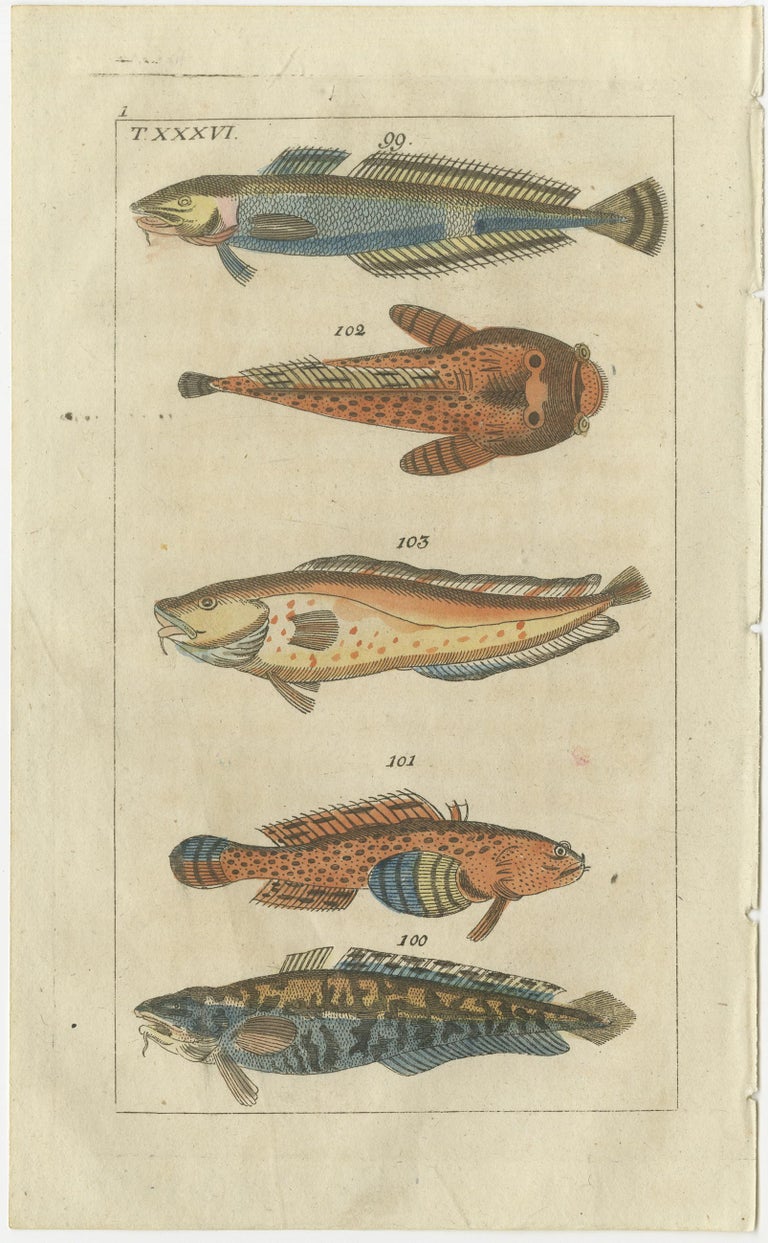This image appears to be a detailed, scientific illustration of five different fish species, set against an aged, brownish-beige paper that resembles a poster. There is a black line border within the paper, about an inch or two from the edge, and the notation "T.XXXVI" is in the top left-hand corner. Each fish is meticulously illustrated with unique color patterns and numbered sequentially from top to bottom: 

1. The top fish, numbered 99, faces left and features a blue body with a yellow head and pink gills, complemented by yellow fins and a tail.
2. Directly below it, the fish number 102 is oriented to the right. This fish is characterized by an orange, catfish-like body with yellow fins and eyes positioned on the top of its head.
3. The third fish, labeled 103, faces left and has a yellow and orange body with orange spots and a hint of blue on its bottom fin. It is shaped more like a bass.
4. Following this is fish number 101, which faces right and boasts an orange body with yellow and blue gills, and fins. Its eyes are distinctively positioned more towards the top of its head.
5. The bottom-most fish is marked with the number 100 and also faces left. It has a larger belly, blue on the bottom, yellow on the top, and is adorned with striped patterns reminiscent of cheetah or zebra prints.

The detailed coloration and positioning of each fish give a comprehensive view, suggesting this illustration could be seen in a scientific context or possibly a decorative piece in a sushi restaurant.